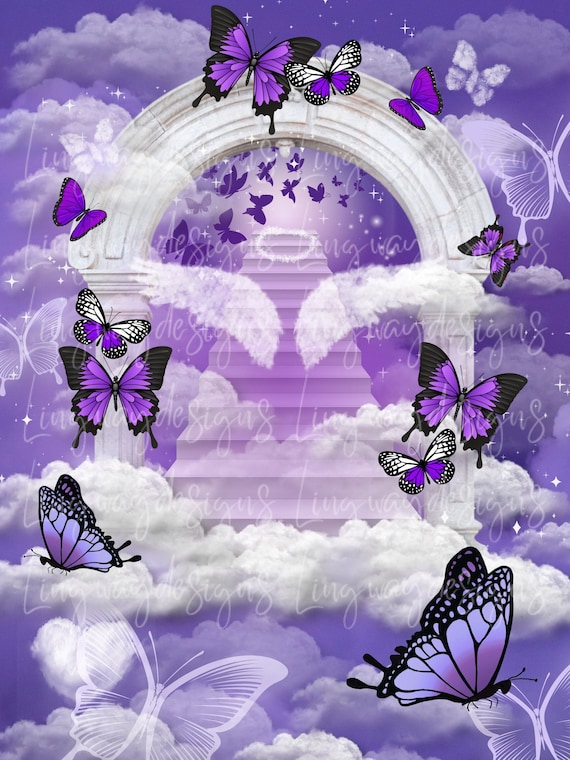This image is a detailed digital painting depicting a fantastical gateway to heaven. The scene is dominated by a grand, concrete archway adorned with delicate ornamentation and sculpting. At the base of this archway begins a white staircase that ascends into a vibrant, purple-hued sky, enveloped in a sea of white clouds. The ethereal atmosphere is further enhanced by numerous purple butterflies, decorated with black swirls along the edges of their wings, fluttering around the entrance and ascending the stairway.

The archway is part of a larger structure supported by pairs of white pillars that connect at the top with a white, bridge-like structure. At the summit of the staircase, a radiant light and a white ring hover, emphasizing the celestial theme. The sky and surrounding ambiance bathed in shades of purple and pink, combined with the clouds and butterflies, creates a dreamy, surreal landscape.

This image is marked with watermarks in a cursive style, though the text is faint and hard to decipher. Among them, "Ling Wei Designs" is visible, suggesting the creator's signature. The image, reminiscent of memorial cards, carries a profound connotation of entering heaven, often seen shared on social media for its evocative, spiritual theme.